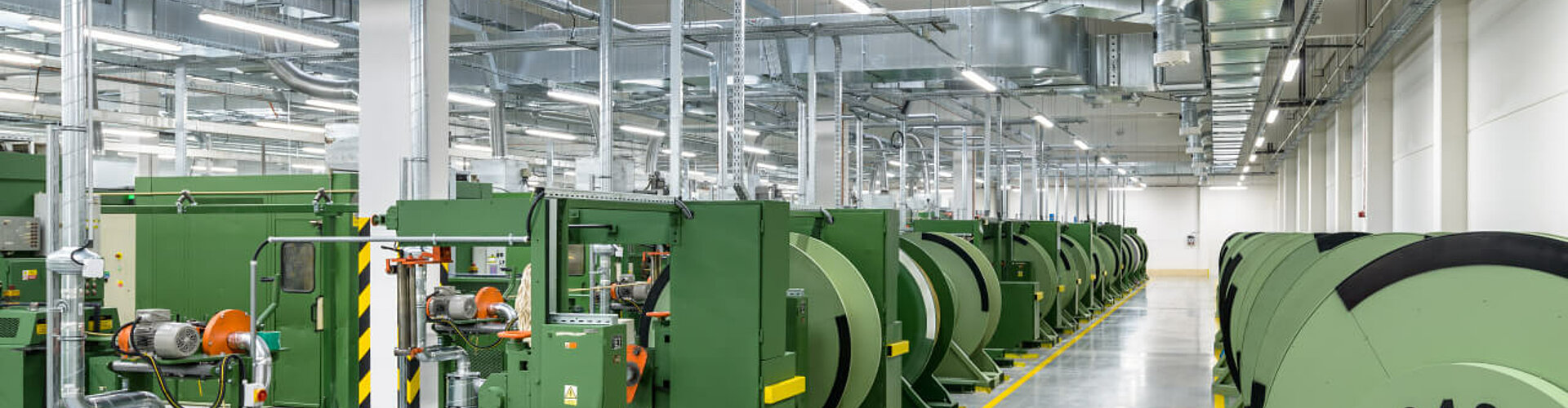The image captures an expansive, wide-angle view of the interior of an industrial facility or factory. The ceiling is crowded with silver metal objects of various shapes, including uneven rectangular and round structures, each reflecting the bright glare from numerous fluorescent lights. The facility’s ceiling is further adorned with an intricate network of metal grid-like frames, vents, and air conditioning units.

At ground level, a shiny gray floor adds a polished, reflective surface to the scene, accentuated by a red painted line that runs along a walkway area near the bottom right corner of the image. On either side of this walkway, several green machines are neatly aligned in a row. These machines, which appear to be complex in design, feature round light green components with black metal or plastic edges. Additionally, there are dark green sections that incorporate orange mechanical parts, further adding to the sophisticated look of these machines. The walls of the facility are stark white, providing a clean backdrop that highlights the industrial landscape.